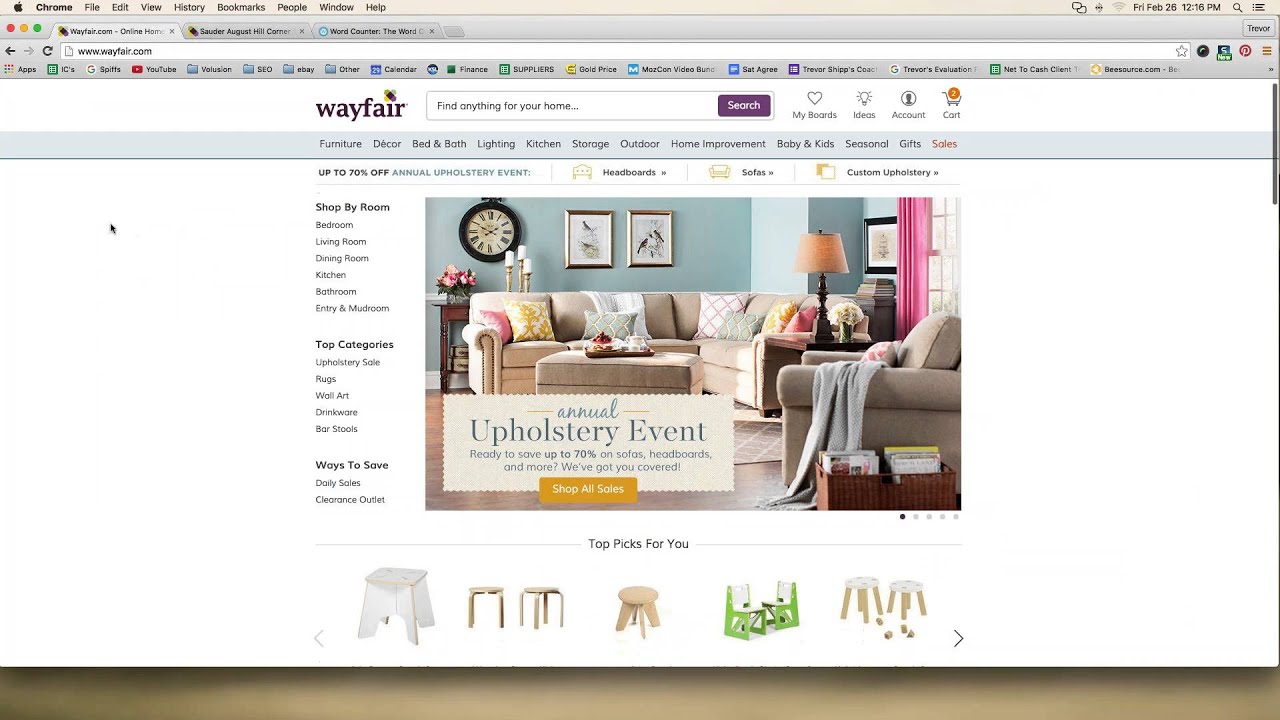**Caption:**

In this PC screenshot, we see the Wayfair.com website accessed through the Chrome browser on an Apple PC, recognizable by its distinct iOS interface elements. The website’s logo, "Wayfair," is prominently displayed in the upper left corner. The main focus of the webpage is a horizontally oriented section taking up most of the middle and foreground, framed by white margins on either side.

The central image showcases a cozy living room with blue walls, featuring a white sectional sofa and a matching chair and ottoman. Pink curtains add a pop of color to the setting. Overlaying this image is a pale blue text banner promoting the "Annual Upholstery Event," encouraging customers to "Save up to 70% on sofas, headboards, and more," with a gold clickable button labeled "Shop All Sales."

Below the living room image are small photos of various types of furniture, such as simple white stools shown from different angles, accompanied by the heading "Top Picks For You" in small dark blue letters, implying that these items were recently searched for.

To the left of the main image, a vertically arranged menu against a white background lists various shopping options in dark blue or black print. Categories include: "Shop by Room" (with subcategories like bedroom, living room, dining room, kitchen, bathroom, entry, and mudroom), "Top Categories" (featuring upholstery sales, rugs, wall art, drinkware, and bar stools), and "Ways to Save" (highlighting daily sales and clearance outlet). This structured layout guides users seamlessly through different sections of the website.